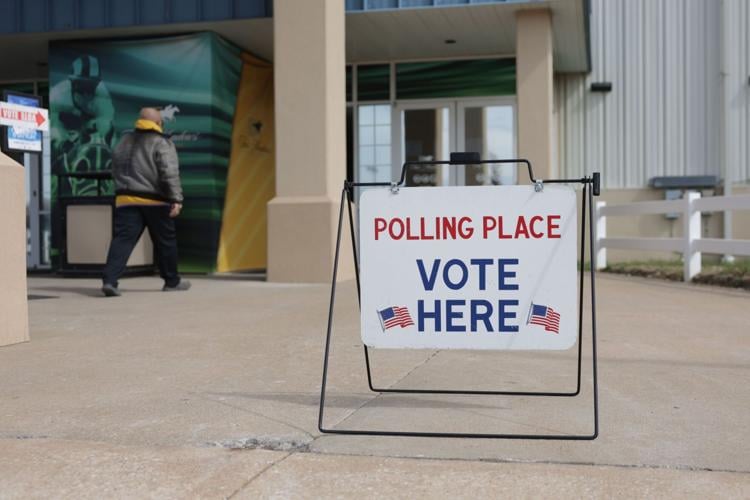The image depicts the exterior of a modern public building, possibly a library or a stadium, with distinct architectural features including vertical white textures, tan concrete columns, and large glass double doors. In the foreground, there is a prominent A-frame metal stand holding a white sign. The sign has "Polling Place" in red letters above "Vote Here" in blue stacked letters, flanked by two American flags. The metal frame is black and rests on a concrete pad. To the right, a white wooden fence runs alongside the building, which also features an image of a cyclist or a person engaging in a sporting activity, adding a decorative touch. Approaching the entrance is a bald African-American man dressed in black pants, gray shoes, a yellow sweatshirt, and a black jacket. He walks towards the glass doors, suggesting he is about to participate in the voting process.